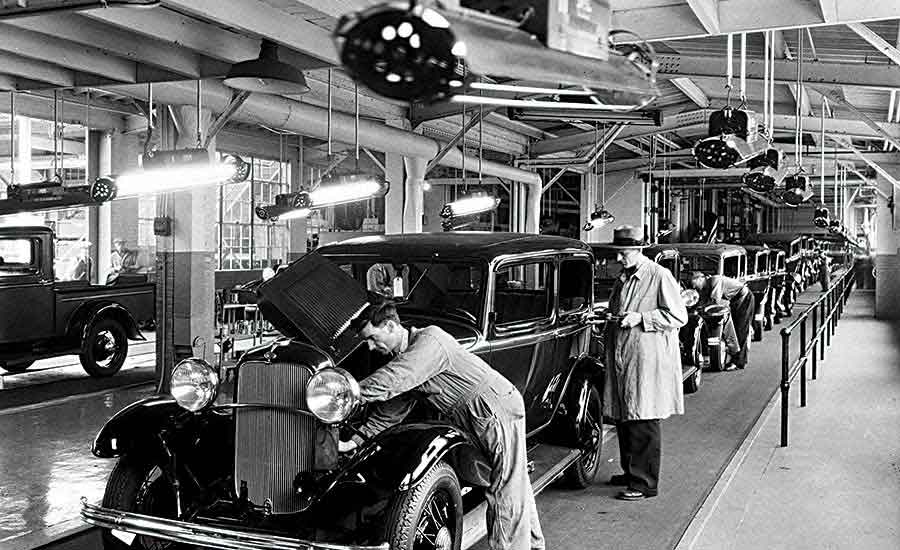This detailed black and white photograph captures a bustling scene in an old automobile factory, likely from the 1920s to 1940s, perhaps even the early 1950s. The image features a long row of fully assembled vintage cars, possibly Model Ts, lined up in the middle of a large warehouse. Overhead lights and an array of pipes accentuate the industrial atmosphere. Mechanics, dressed in jumpsuits, are seen bent over the hoods of the cars, tuning up the engines. Amidst them, a distinguished man in a coat, slacks, dress shoes, and a hat, possibly an inspector or supervisor, walks through the assembly line with a clipboard, likely running a checklist inspection. The backdrop reveals additional workers and various factory elements, including a sidewalk-like pathway with a gate and another old car by the wall. The scene evokes the early days of American automotive production, highlighting the meticulous process and the organized assembly line that revolutionized the industry.